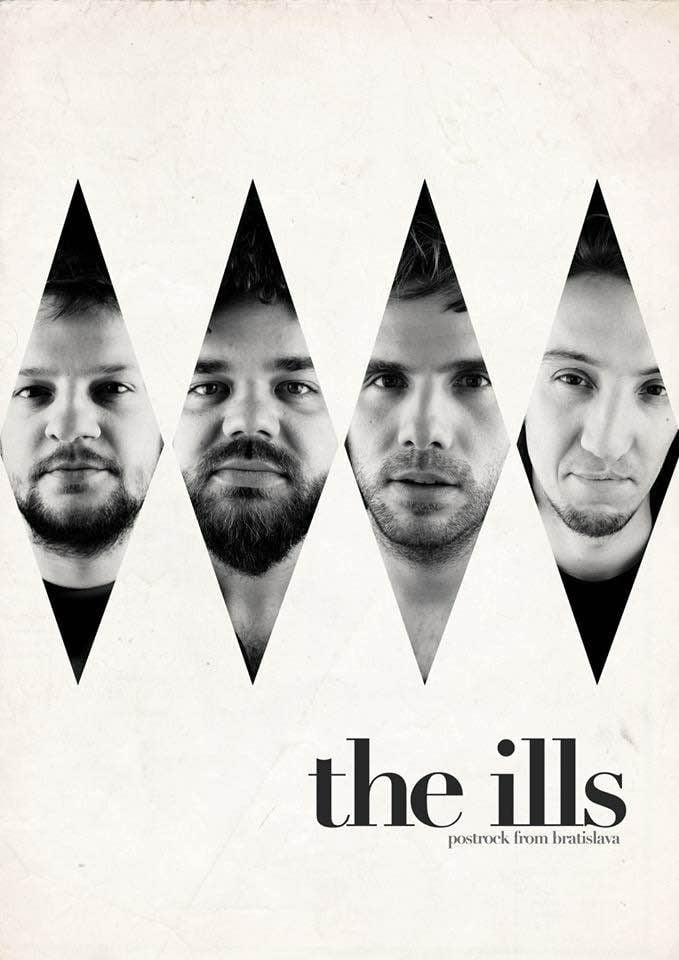The poster for the band "The Ills" is designed with a textured white background that mimics the look of old, slightly dingy paper, complete with artifacting and a fold running from top to bottom. The band name "The Ills" is prominently displayed in lowercase serif font, with the phrase "Post Rock from Bratislava" inscribed in much smaller letters underneath. The central feature of the poster comprises four elongated diamond-shaped, black-and-white photographs that span across the middle of the graphic. Each diamond houses the face of a bearded male band member, with varying styles of facial hair ranging from a tiny goatee to a fuller beard and mustache. The men are all staring directly at the camera, with the diamond shapes partially cropping their faces. This composition suggests a focus on the band's unique identity and stylistic coherence.